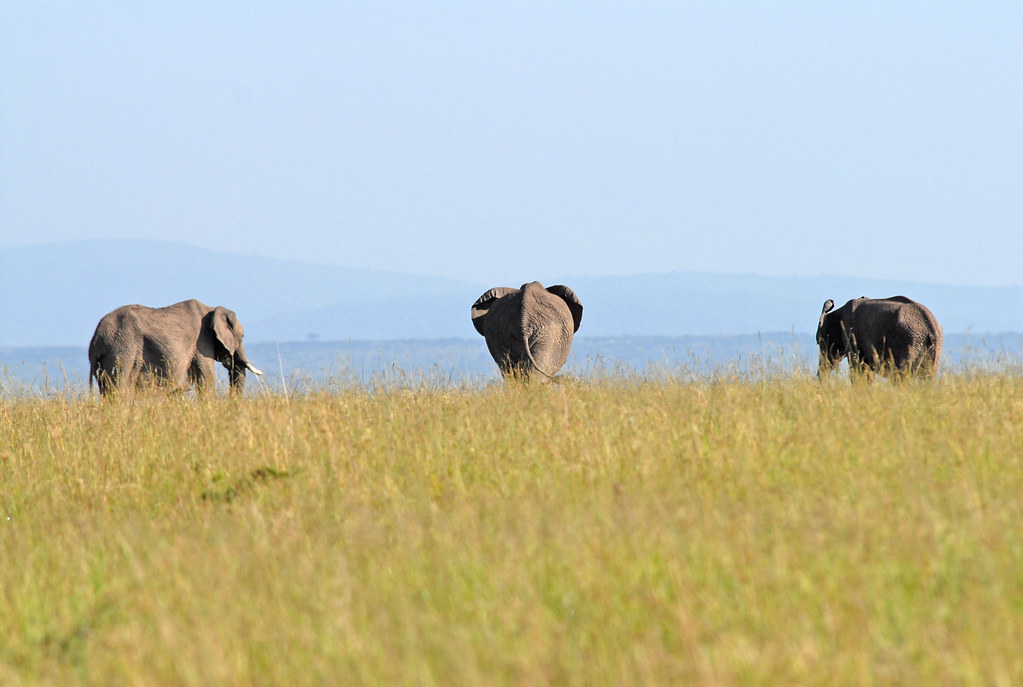This vibrant outdoor daytime scene captures three majestic, full-grown elephants walking through a field of tall, greenish-brown grass in the African grasslands. The elephants are spaced equidistantly, heading away from the photographer, with their large ears, long trunks, and formidable tusks prominently visible. The grass appears fine and somewhat dry, adding texture to the image. In the deep background, a hazy blue mist cloaks distant hills or mountains, creating a serene contrast against the lighter sky above. The elephant on the left has conspicuous tusks approximately a foot long, while the one in the center displays its tail and large ears. Despite the peaceful ambiance, the elephant on the right looks slightly malnourished. The overall scene is devoid of clouds, and the photograph's composition beautifully captures the essence of the elephants in their natural habitat.